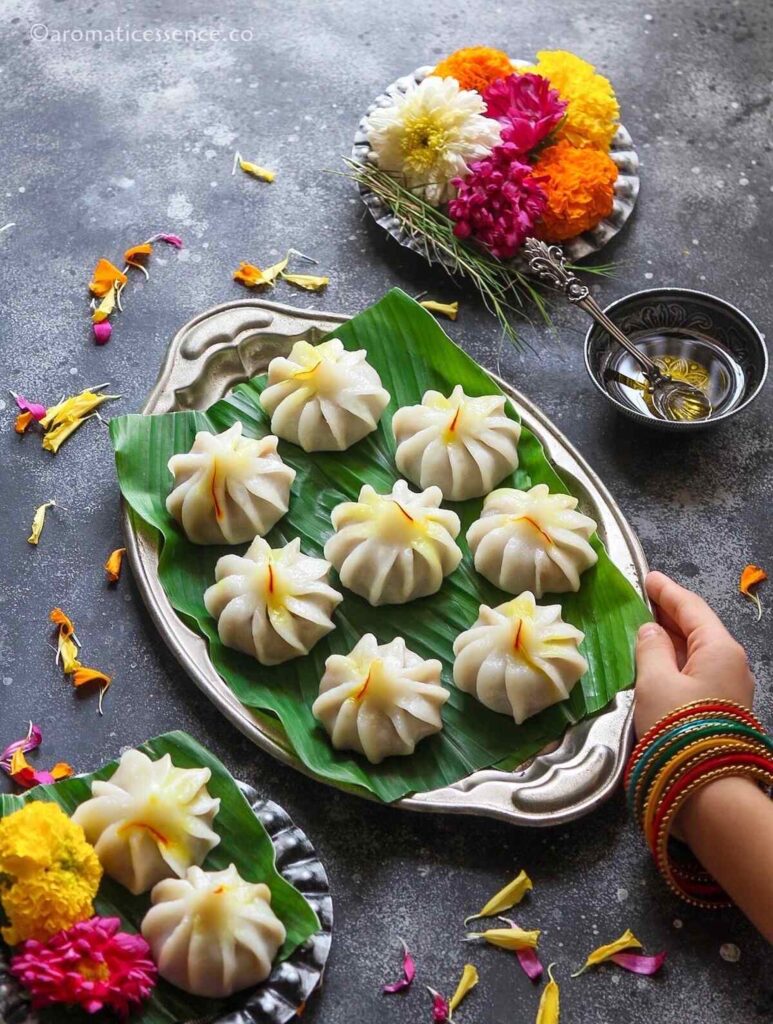This photograph, credited to aromaticessence.co, showcases a beautifully arranged plate of white dumplings with saffron threads on a green leaf, placed on a steel oblong platter at the center of the image. The platter is held by a hand adorned with multiple colorful bangles, likely belonging to the person who made or served the dumplings. Surrounding the central plate are scattered multicolored flower petals, enhancing the vibrant aesthetic. To the right is a small silver bowl with a spoon, containing a clear syrup with a yellow tint. At the top of the image, a small silver plate holds five flowers, adding an extra touch of elegance. In the bottom left corner, another small plate features two similar dumplings on a green leaf, accompanied by three flowers, all set against what appears to be a marble or concrete surface.